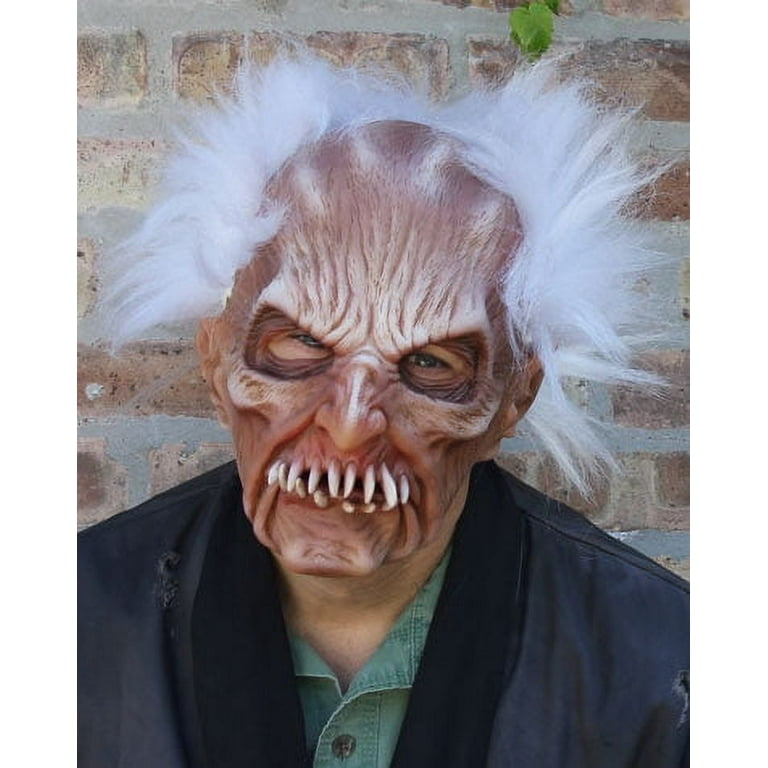A man stands against a brick wall with gray cement between the bricks, wearing a dark blue jacket with a blue jean texture and a light green, button-up shirt underneath. His face is covered by a striking and ominous mask reminiscent of a ghoul's visage. The mask features a long, hooked nose with a white stripe running down its center. The mask has thick, white hair sprouting wildly in all directions from its mostly bald top, with wrinkles and an area of white just above the eye openings. The eye openings narrow at the front and widen at the outer edges, revealing the man's light blue eyes set behind the mask. The mask's skin is reddish, with fierce, white, claw-like teeth protruding menacingly both from the top and the bottom of the mouth, which lacks lips. The teeth at the bottom appear slightly dirtier and more worn. The overall effect is eerie, with detailed wrinkles adorning the sides of the mask’s chin, enhancing its lifelike horror.